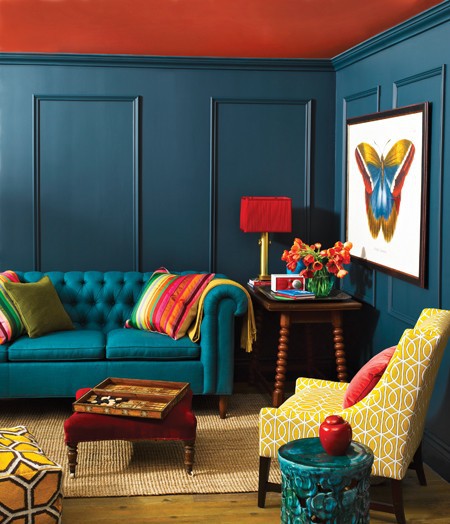This full-color photograph captures a vibrant living room interior. The room features a distinctive combination of bright red, smooth-painted ceiling and walls in a lively blue or dark teal hue, adorned with oblong grid patterns and crown molding for added dimension. The floor is wooden, showcasing visible knots, and it is partially covered by a rug.

Prominently positioned on one of the walls is a large, framed painting of a colorful butterfly with a white background, adding a focal point to the decor. Below the painting sits a turquoise couch, detailed with button-tufted divots and covered in a colorful, rainbow-hued blanket and pillows. Adjacent to the couch is a wooden table with intricately designed, spool-like legs, holding a red lamp with a gold base and a bouquet of flowers.

A yellow chair with white, giraffe-like patterns stands out in the room, complemented by a red pillow. Additional furnishings include a blue table topped with a striking red jar. The eclectic mix of colors and patterns throughout the space creates a visually stimulating and cheerful ambiance.